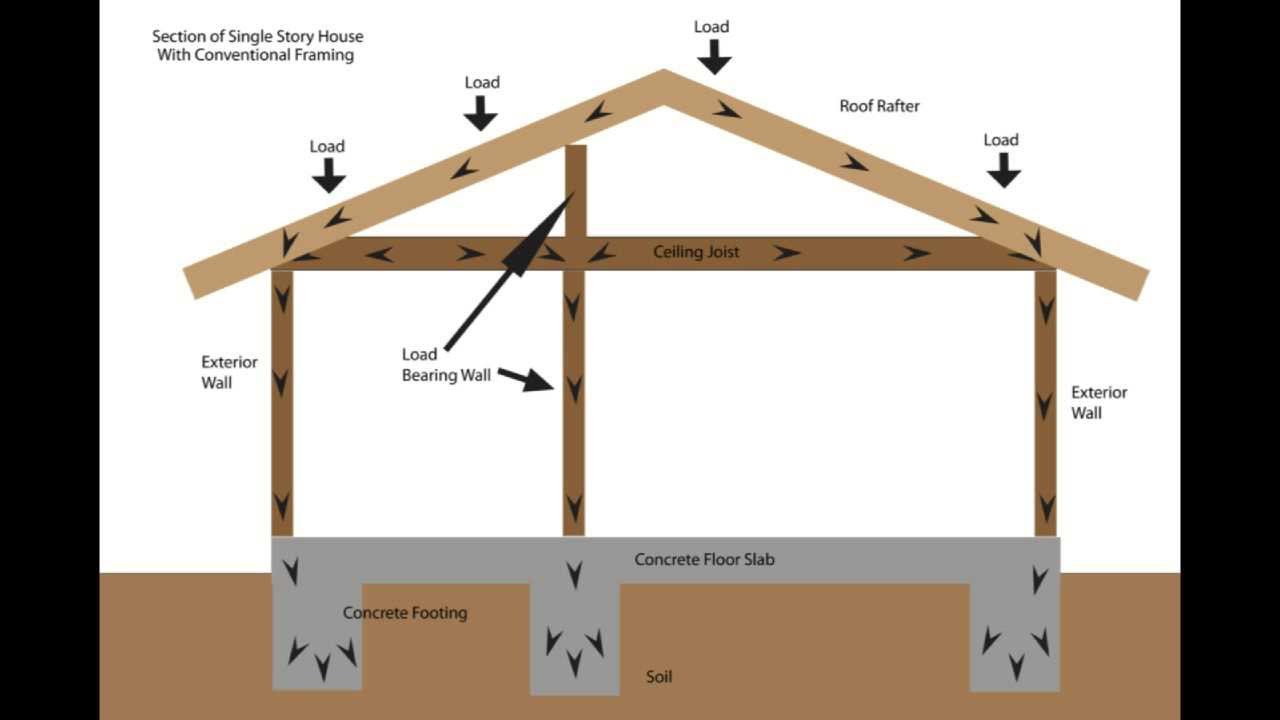The image depicts a detailed section cut diagram of a single-story house with conventional framing, as seen on a web page or from a PowerPoint presentation. The main background of the image is white, while the bottom quarter is brown, indicating the ground. Labeled components include the soil, concrete footings extending into the ground, and the concrete floor slab. The basic wooden frame of the house is illustrated, including the exterior walls, a centralized load-bearing wall, ceiling joists, and roof rafters. The roof is shown in a side view with black arrows indicating the load-bearing areas of the beams and the roof. The diagram is minimalistic, with clear labels and directional arrows highlighting crucial structural elements such as the concrete footing, wall framing, and load distribution.